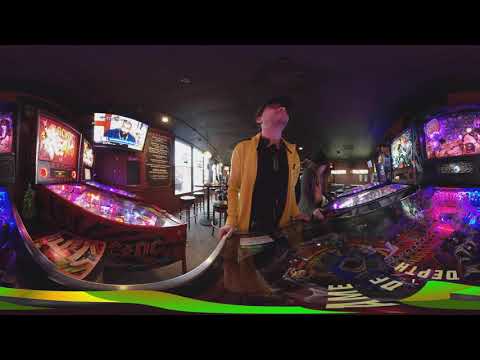In this photograph set in a dimly lit pinball alley, a man stands in the center, surrounded by an array of illuminated pinball machines emitting vibrant pink, purple, blue, orange, and yellow lights. He is dressed in a yellowish-brown jacket over a black shirt, his outfit accented by a black golf cap. The man gazes dramatically upwards, seemingly uninterested in the pinball machine he’s playing. 

Behind him stands a woman, engrossed in her own pinball game. She wears an olive cardigan over a pink shirt and also sports a cap. The left side of the image features a line of windows letting in some light, below which hangs what appears to be a menu on the wall. A television screen is mounted nearby, further left, partially visible. 

The ceiling overhead is dark, with light filtering in from distant windows, illuminating stools and tables along the periphery. The photograph has black bands across the top and bottom, adding to the focus on the dramatically lit central figures—the man in his distinctive jacket and the woman in her cardigan.